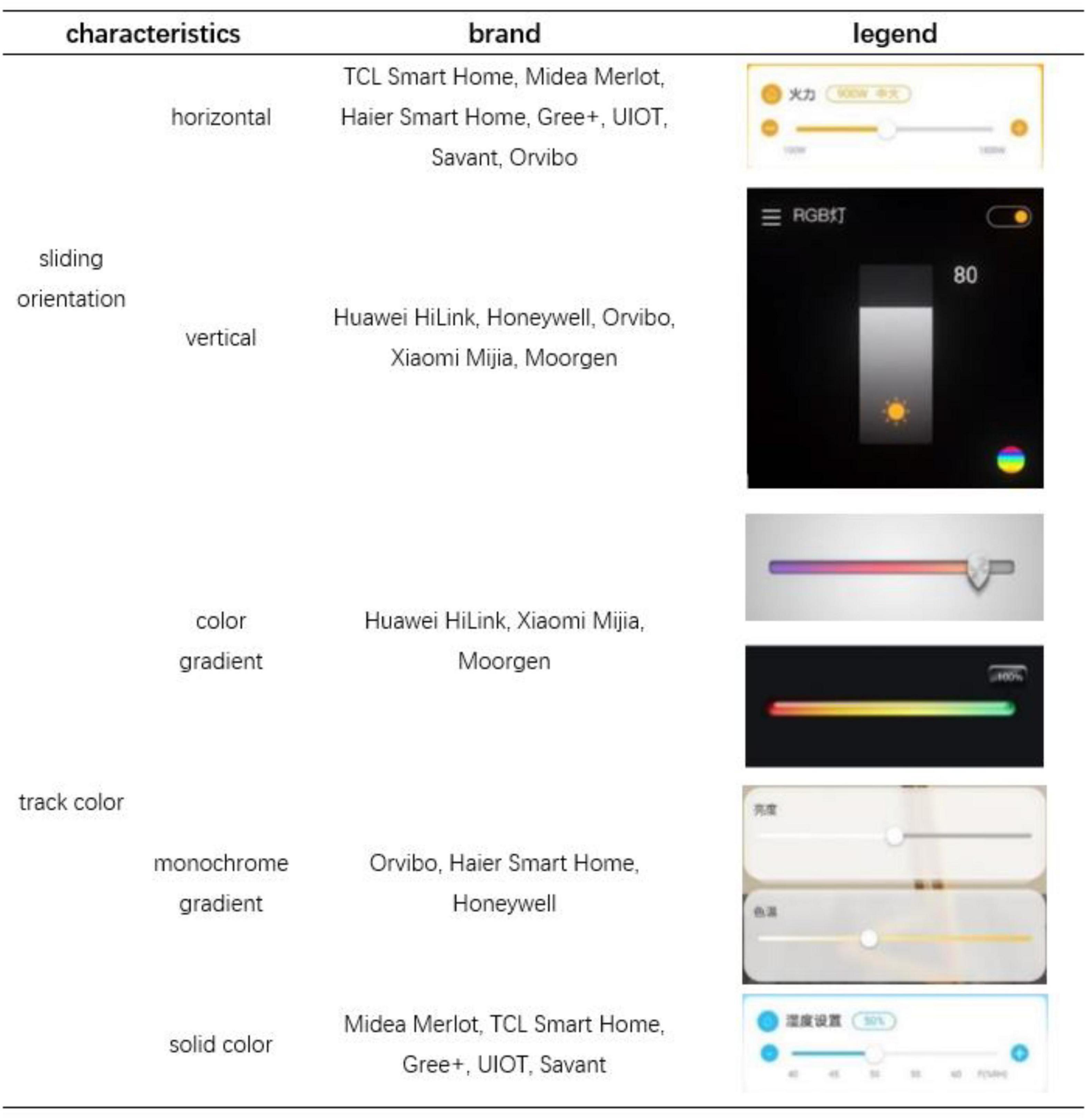The image depicts a detailed chart against a white background with black text. Along the right-hand side, several images are arranged vertically, complementing the chart. The chart itself is divided into three sections, labeled "Characteristics," "Brand," and "Legend."

Adjacent to the headings, four main images provide visual context:
1. **Top Image:** A black box containing a gray rectangle with an orange sun shape at the bottom. In the upper right-hand corner, the number "80" is displayed. Below the rectangle, there is a circle featuring horizontally colored stripes.
2. **Second Image:** A gray rectangle topped with a multicolored horizontal bar accompanied by a gray, knob-like figure.
3. **Third Image:** A black box showcasing a rod colored in rainbow hues.
4. **Bottom Images:** Two grayish rectangles. Each rectangle has horizontal lines with a single white disk positioned in the middle.

The descriptive and visual elements combine in this meticulous chart to illustrate the "Characteristics," "Brand," and "Legend" related to the provided visual data.